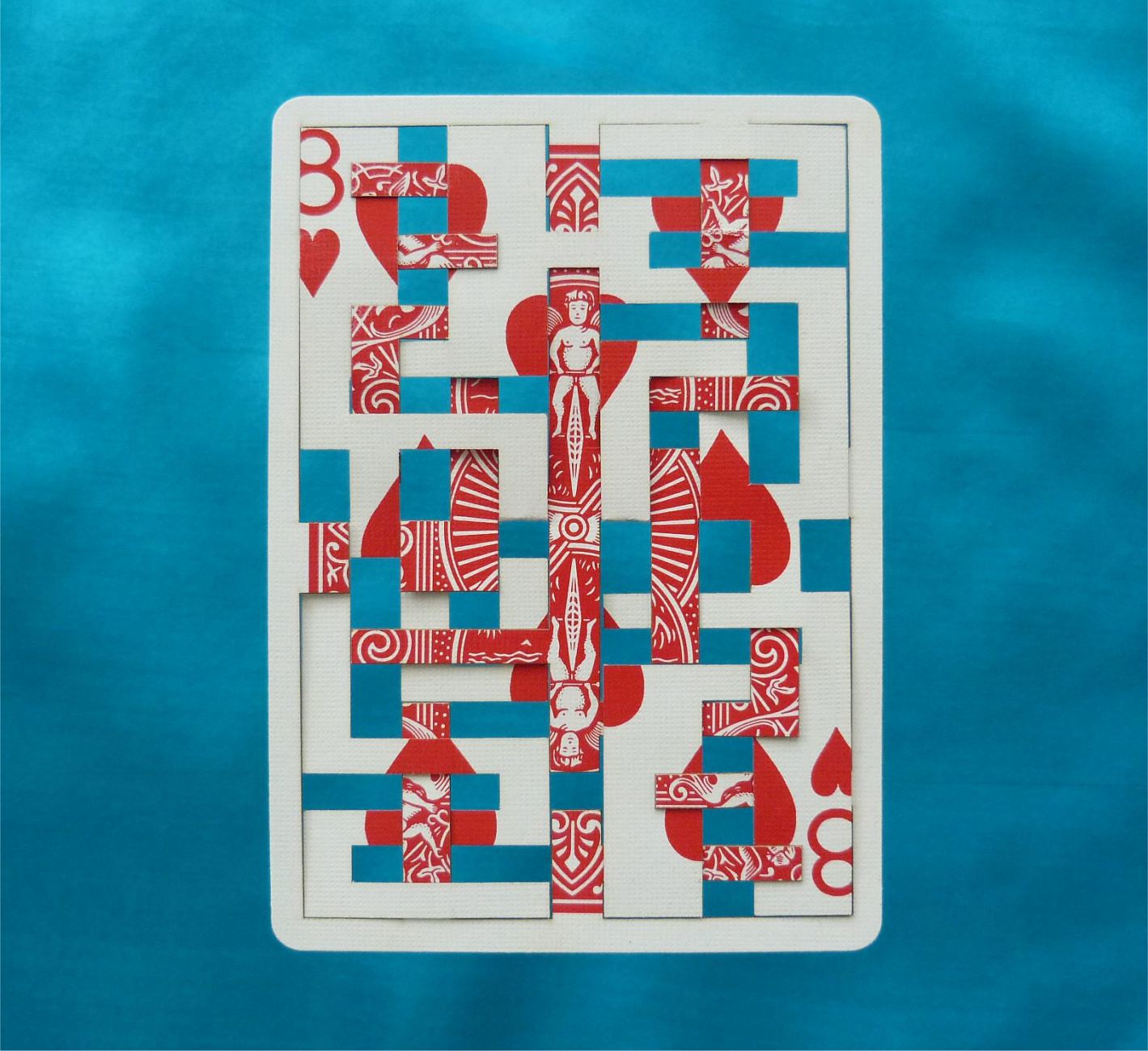A highly intricate photograph showcases a creatively manipulated playing card, meticulously cut and reassembled in an origami-like fashion. The card, an eight of hearts with a white background and classic red markings, rests on a richly textured turquoise fabric. The fabric’s gradient blend from a darker turquoise at the bottom to a lighter shade at the top adds depth and contrast to the scene.

The playing card itself is a rectangular shape with rounded edges, featuring an intricate cut-out design. Inside the main rectangle of the card, various smaller rectangles and triangles have been excised and repositioned to overlap each other, forming an elaborate pattern. The interplay of the reassembled pieces exposes fragments of the card’s design, including bits of red hearts, segments of cherubs, and parts of the circular motifs typically found on playing cards. The top left and bottom right corners prominently display the red number eight and heart symbol, anchoring the viewer’s eye amidst the complex arrangement. The overall composition is a harmonious blend of traditional card elements and abstract artistic expression.